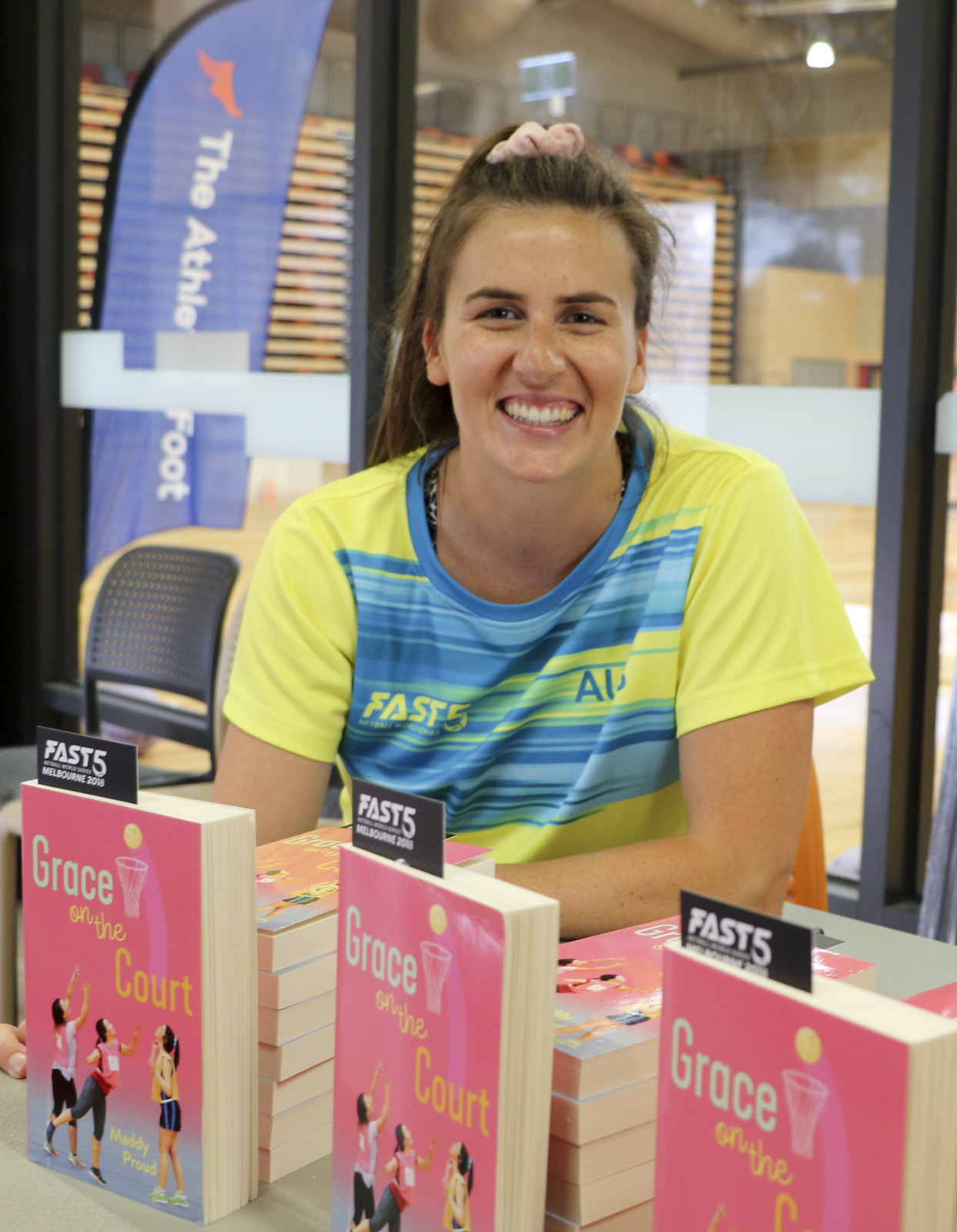The landscape-oriented color photograph depicts a lively book signing event at an Athlete's Foot store in a mall, with emphasis on the details of both the subject and the setting. At the center of the image is a young woman, identified as Maddie Proud, smiling broadly at the camera. Her straight, long brown hair is partially pulled back with a pink scrunchie. Clad in a yellow and blue striped jersey, which also has shades of green, she exudes enthusiasm and charisma. Maddie is leaning forward with both elbows resting on a table, around which stacks of her book, "Grace on the Court," are arranged. The book covers, primarily pink with a depiction of three girls playing basketball and a title clearly visible, add a splash of color to the scene. Notably, the book includes a tag indicating "Fast Five Melbourne 2018." Behind Maddie, glass doors open into the gym-like store space, where a vertical banner featuring the athlete's foot logo in red against a blue background is prominently displayed. The scene captures Maddie's dual identity as both an athlete, given her Fast Five shirt, and an author, while the mall setting provides a bustling, energetic backdrop, complete with visible shops through the windows.